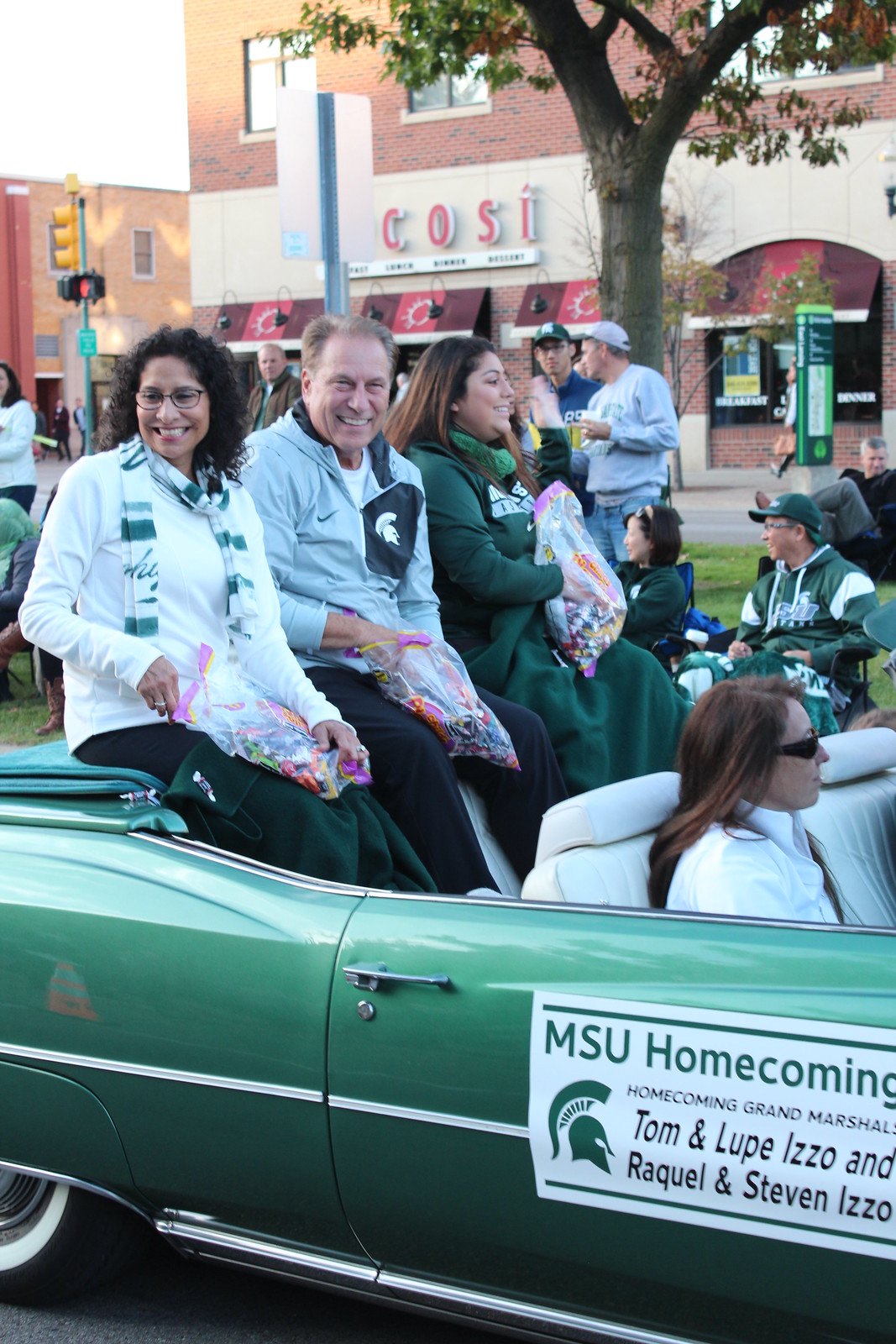The image depicts a lively MSU Homecoming parade taking place on a sunny afternoon, casting long shadows on the street. Central to the scene is a classic green and white 1950s convertible, likely a Corvette, carrying the Homecoming Grand Marshals, Tom and Lupe Izzo along with Raquel and Stephen Izzo. The occupants, consisting of two women and one man, are seated on the back of the car, engaging enthusiastically with the parade crowd by throwing candy from a bag. The woman on the left wears a white sweater paired with a green and white striped scarf, while the woman on her right is dressed entirely in green. In the passenger seat, another woman with long brown hair and sunglasses complements the festive spirit. The backdrop features a downtown setting with various buildings, notably a restaurant named "C-O-S-I," and a traffic light, enhancing the vibrancy of the event. Many onlookers, also clad in MSU colors of green and white, line the parade route, framed by the intersection and storefronts, celebrating the Michigan State University Spartans.